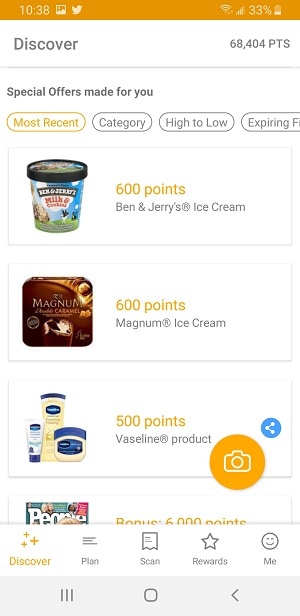This image is a screenshot of what appears to be an Android phone interface. The top of the screen features a long orange heading bar. On the left side of this bar, the time is displayed as 10:38, followed by a picture icon and a bird icon. On the right side, there are several status icons: a Wi-Fi icon, signal bars indicating nearly full strength, and a battery icon showing 33% charge.

Below the heading bar, there's a text on the left-hand side that reads "Discover," and on the right-hand side, it says "68404pts." A thin line separates this section from the rest of the screen.

The next section contains options presented in oval buttons: "Special Offers Made for You," "Most Recent," "Category," "High to Low," and "Expiring." The "Most Recent" option is highlighted. 

Following this, the screen displays various products and their corresponding point values, starting with an image of Ben & Jerry's ice cream, which costs 600 points. Next to it is an image of Magnum ice cream, also priced at 600 points. Below that, there's a Vaseline product worth 500 points, accompanied by a picture and an overlay icon of a camera. There is also a share button within the Vaseline section on the right.

Finally, partially visible at the bottom of the screen is what seems to be an image of People magazine and some additional icons.